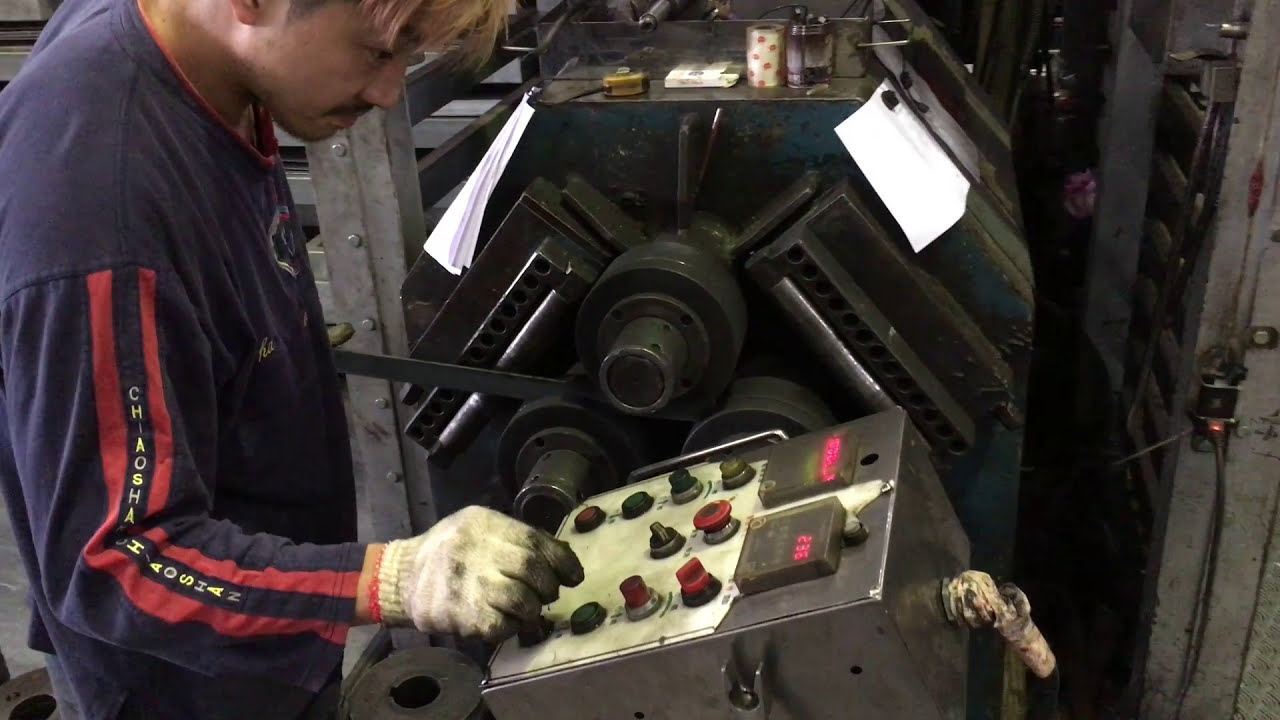In this detailed indoor scene, an Asian or South Asian man is standing on the left side of the frame in a mechanical facility, engaging with a control panel in front of him. The control panel features various red, green, and black indicators and buttons, including emergency stop buttons and dials displaying red numbers. The panel is connected to a larger piece of machinery with multiple shafts and intricate components, including double-layered metal blocks, white conduits, and a silver frame extending to both sides.

The man, who has dark brown razor-burned facial hair and dyed blonde and light pink hair, is dressed in a navy blue long-sleeve t-shirt with prominent red stripes along the neckline and sleeves. The shirt bears the text "Chiao Sha" or "Kiao Sha," seemingly a Chinese company name or logo. He is also wearing wool gloves, heavily soiled with grease, and a red item is visible around his wrist beneath the gloves. The environment is cluttered with various tools and mechanical apparatus, reinforcing the industrial ambiance. The color palette in the image includes shades of blue, red, white, yellow, brown, teal, and purple.